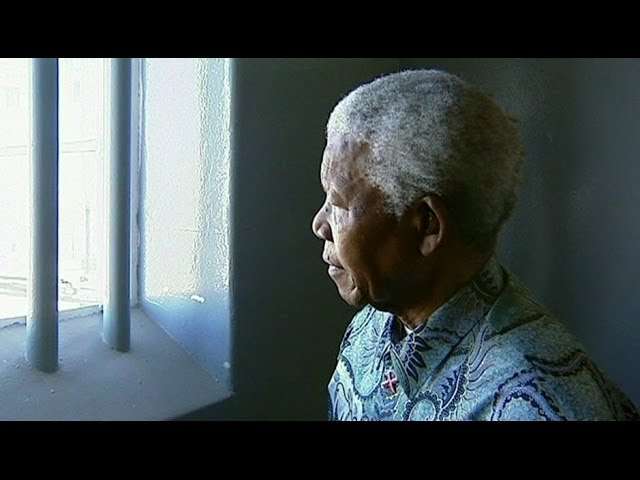This is a detailed photograph of Nelson Mandela in a prison cell, capturing the left side of his face and extending down to his shoulder. He is sitting beside a barred window, with two gray bars casting shadows. The wall behind him is also gray, adding to the somber atmosphere. Mandela is wearing a light blue shirt adorned with a dark blue and white pattern, possibly paisley, with distinctive buttons that have an "x" on them. His hair is gray, and a small mole or wart is visible on his nose. The light outside reflects off the wall beside the window, illuminating his thoughtful and curious expression. Despite the muted color palette, Mandela's serene demeanor stands out, creating a powerful and emotive image.